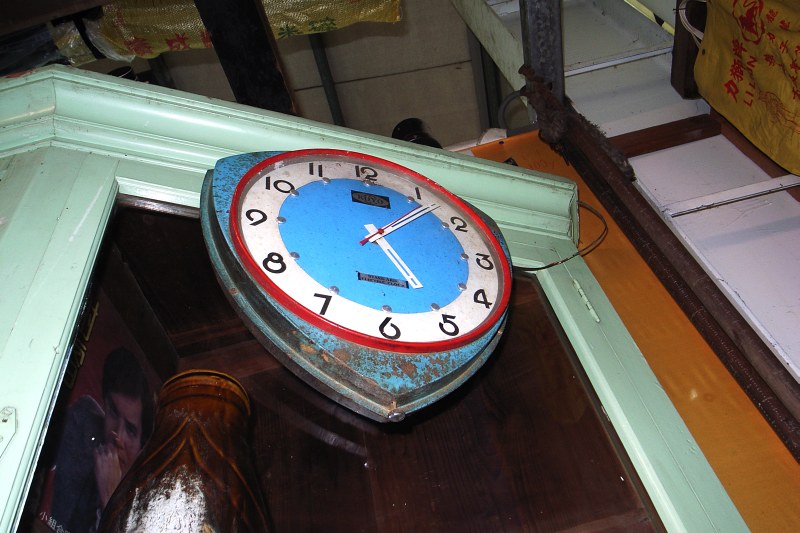The image captures an upward perspective of a wall-mounted clock situated on a green dish hutch inside a home. This hutch features a glass door, through which a vase can be seen in the background. The clock itself is designed like a shield, with a rusted exterior. The clock face alternates between blue and white, and includes a red line marking the start of each hour. The clock reads approximately 5:07, with white hour and minute hands, and a red second hand. The numbers on the clock are black, each accompanied by small silver dots. The ceiling of the room is also visible in the frame.